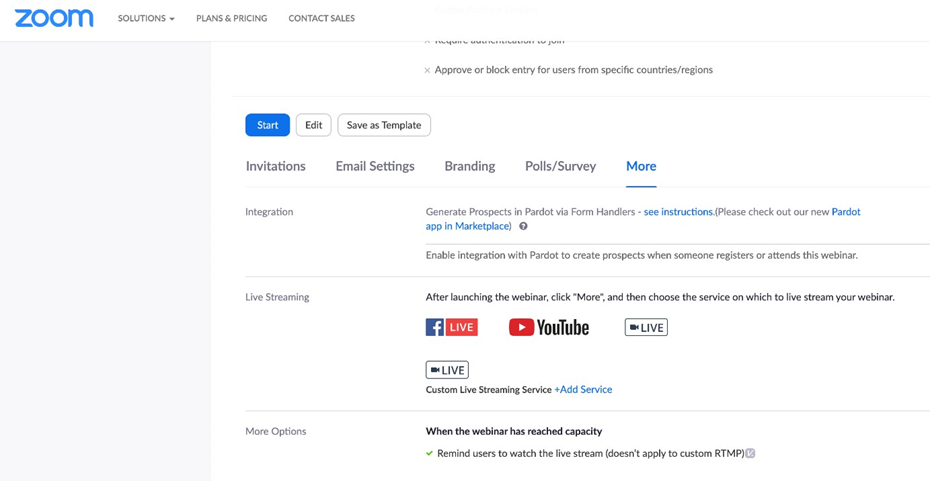The image is divided into two distinct sections. On the left, a light gray area features a navigation menu at the top that includes the options: "Zoom," "Solution," "Plan," "Pricing," and "Contact Sales." On the right, a white space provides a series of actions and settings beginning with the instruction to "Approve or block entry for users from specific countries or regions." 

Below this, there are actionable buttons: a blue "Start" button, a white "Edit" button, and a white "Save as Template" button. Following these buttons are additional menu options including "Invitation," "Email Setting," "Branding," "Poll Survey," and "More."

Further down, a line separates these options from the "Integration" section, which advises: "Generate prospects in Pardot via form handler, see instruction." It also has a note encouraging users to "Please check out our new Pardot app in Marketplace."

Another line introduces the "Enable Integration with Pardot to create prospects when someone registers or attends this webinar." 

Continuing below this, a third line segment indicates instructions for "Live Streaming," suggesting: "After launching the webinar, click 'More' and then choose the service on which to live stream your webinar."

Finally, under the "More Options" heading, it notes: "When the webinar has reached capacity, remind users to match the live stream."